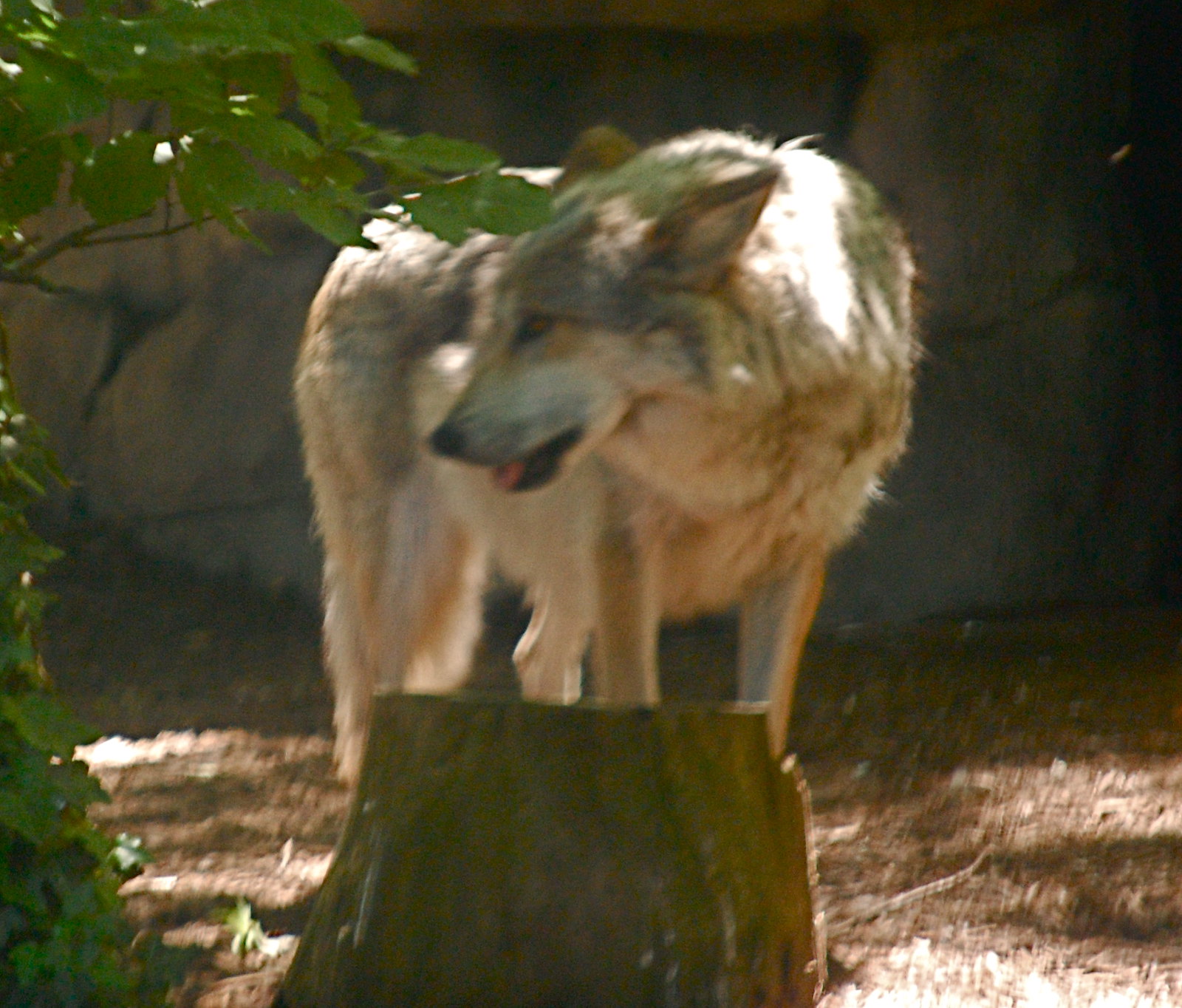This is a detailed close-up photograph of a coyote, characterized by its brown and gray fur. The coyote's ears are slightly pinned back, giving an impression of apprehensiveness, and its snout is turned to the left, not directly facing the camera. Its tongue is out, hinting at the likelihood of hot weather, enhanced by the golden hue of light bathing the scene. The setting appears to be controlled, such as a zoo or a wildlife rehabilitation center, rather than a wild habitat. Behind the coyote, there is a substantial rock wall, adding to the enclosure-like atmosphere. On the left side, a carefully positioned green leaf and a tree stump are visible. The ground is covered with dirt, bark, and debris, indicating a naturalistic enclosure. The overall environment is bright and clear, benefiting from ample natural daylight.